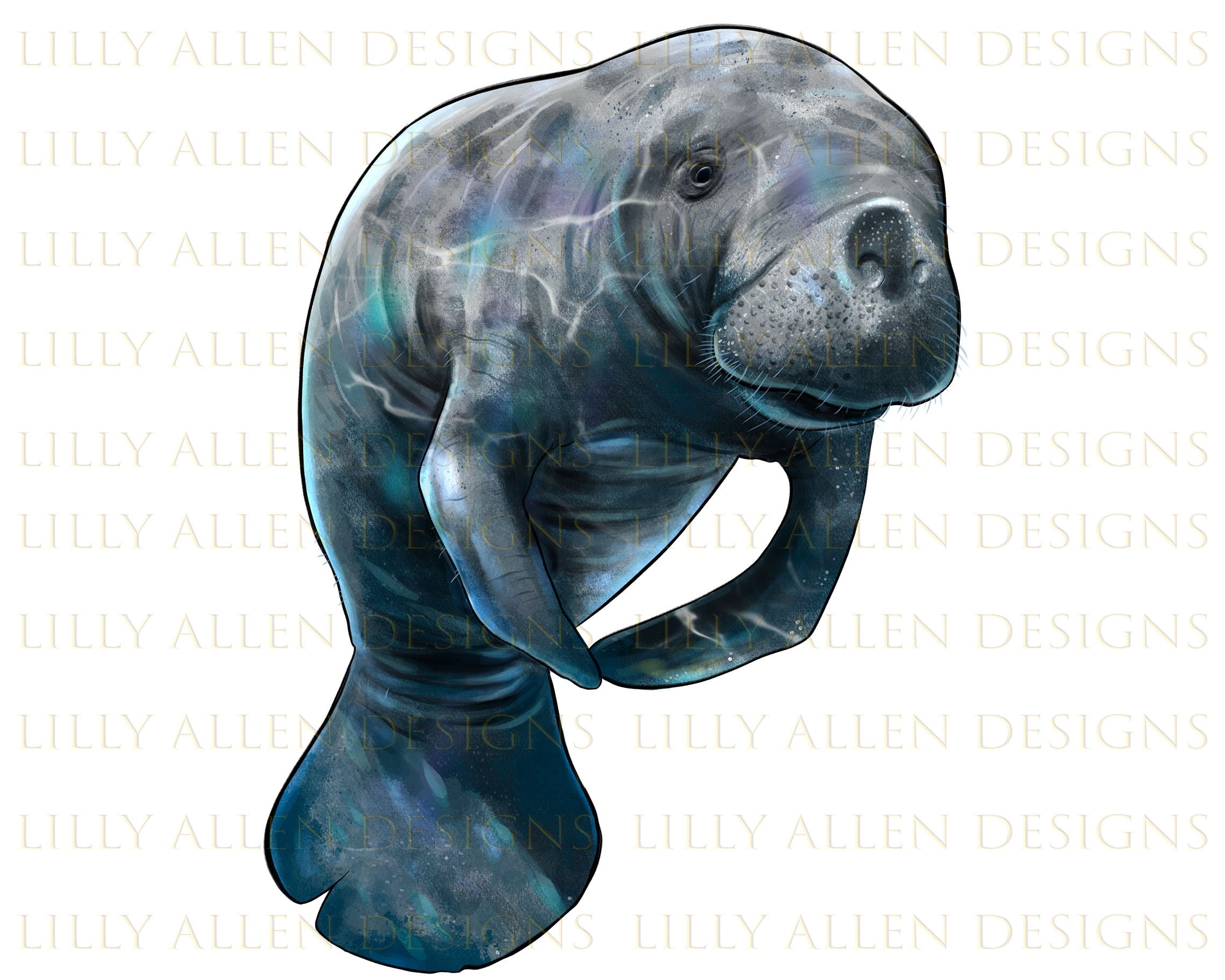This is a detailed and artistic drawing of a manatee, rendered in shades of medium and dark gray with light blue and white reflections that give it a speckled, lifelike appearance. The manatee is positioned centrally on a stark white background, facing toward the camera with its head slightly tilted to the left. Its large, whiskered snout and small eyes are prominent, and its mouth is barely open. The manatee's flippers are pulled together in front of its body, giving the impression that it might carry something. Its tail, which has a small nick, points downward, enhancing the floating effect. The entire image is outlined in black, which adds to the drawing's clarity. Across the background, the watermark "Lily Allen Designs" repeats in light gray text, fading slightly from top to bottom, lending an artistic proof feel to the piece.